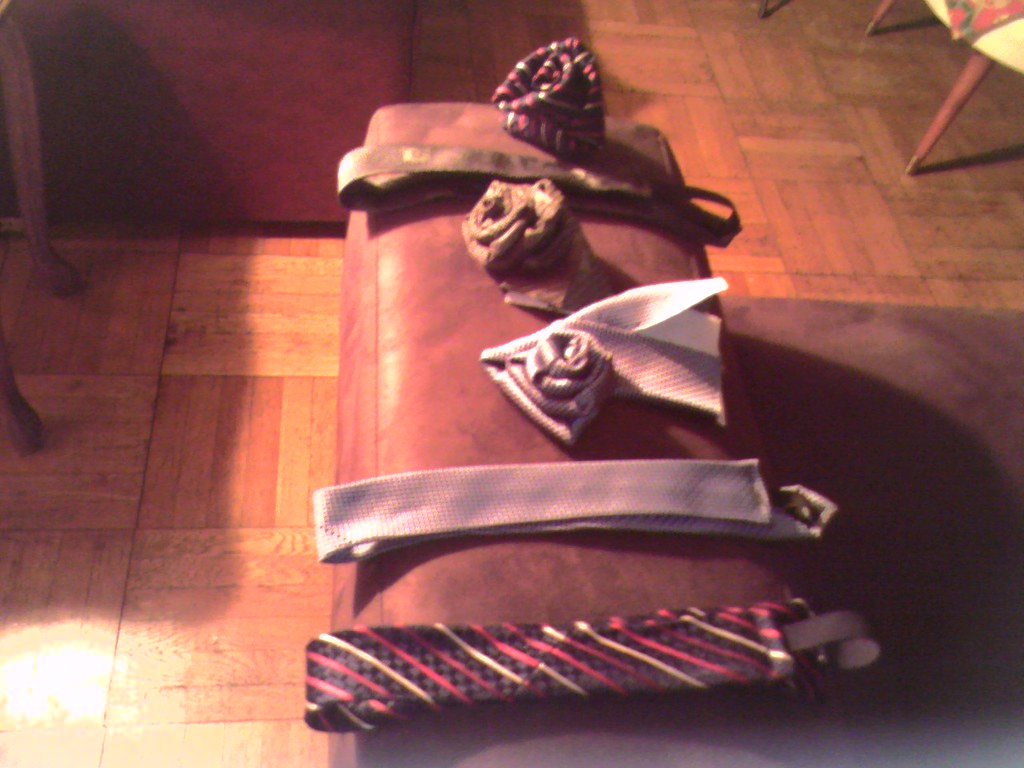In this slightly blurry, horizontal rectangular color photograph, an assortment of men's neckties and rosettes are displayed on the arm of a burgundy couch, with a wooden floor visible in the background. The ties are arranged horizontally along the vertical cushion of the couch, each showcasing unique patterns and colors. The bottom tie is black with red and perhaps yellow or white diagonal stripes. Above it, an upside-down tie features a light pattern, and next to it is a rosette, possibly made from the same fabric. A golden-brown rosette lies beside a matching brownish-gold tie, followed by another rosette of similar material. The arm of the couch, adorned with these ties, is situated within a cozy indoor setting, as suggested by the small table with yellow tabletop visible to the right. The floor, made up of square sections of wooden planks arranged in varying directions, adds a warm touch to the scene. Additional furniture, similarly colored in shades of reddish or brown, occupies the upper left corner, while the chair legs, orangish in color, and the partial view of a yellow chair, add context to the homely backdrop. Natural light streams in from the lower left-hand corner, casting reflections and shadows across the room.